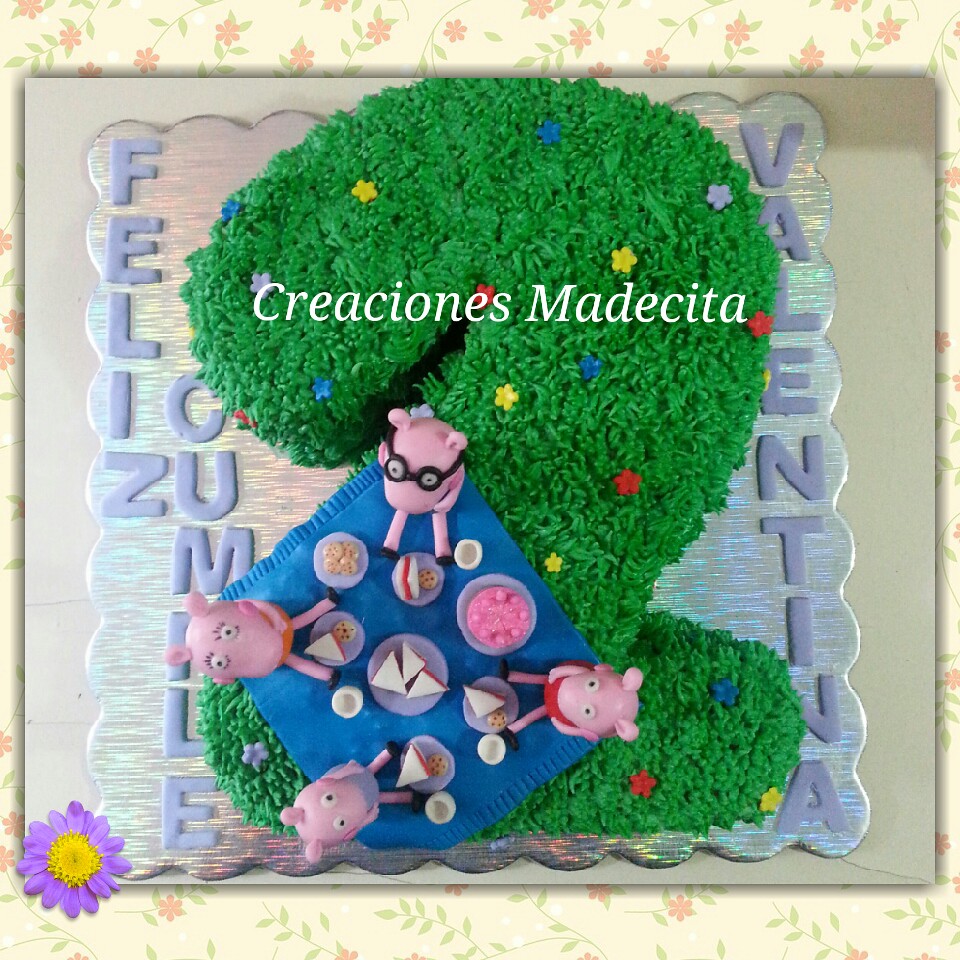This image depicts an elaborate, Spanish-language birthday cake for a child's second birthday, themed around Peppa Pig. The cake, shaped into the number 2, is decorated with green icing styled to look like grass, complete with an array of small candy flowers in yellow, blue, red, and purple. 

Positioned at the lower left of the cake is a fondant picnic scene featuring the entire Peppa Pig family. The family, including Peppa in a red dress, her sibling in a purple dress, their mother in an orange dress, and their father with glasses, is seated on a blue picnic blanket. They are enjoying a picnic with sandwiches, cookies, and a small pink cake. 

The cake is displayed on a silvery, rainbow-shimmer platter, which rests on a gray plate. Surrounding the cake, the border includes floral decorations with pink flowers and green leaves. Text in light blue fondant letters spells out "Feliz Cumple Valentina" vertically along the sides, and a watermark "Creaciones Madecita" overlays the center upper part of the image. A purple flower with a yellow center adorns the lower left corner of the plate.